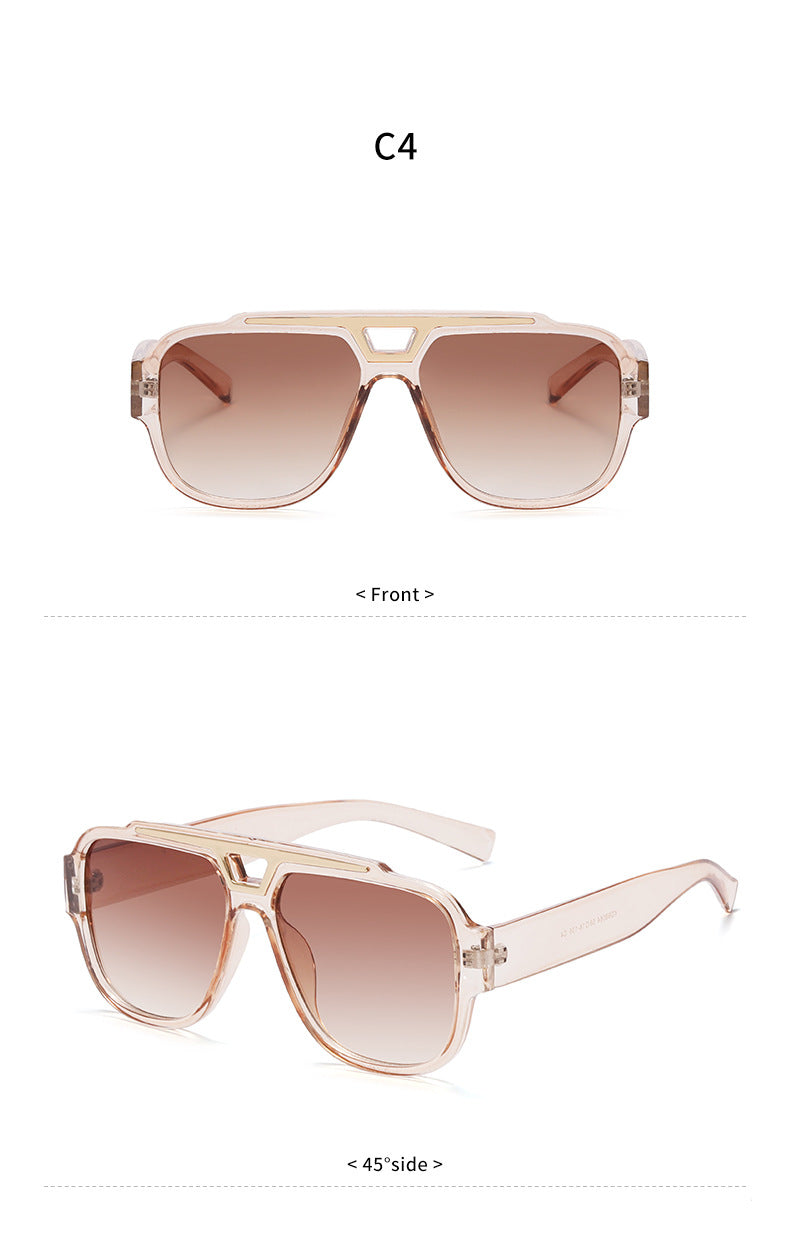This image features a pair of modern, plastic sunglasses depicted in a catalog or sales ad, showcased against a white background. The sunglasses have a light tannish brown frame with a hint of rose-gold shimmer, and the lenses exhibit a gradient from a darker shade at the top to a lighter shade at the bottom. The frame combines square and rounded elements for a contemporary look, and the arm pieces are thicker, ensuring durability.

There are two distinct views of the sunglasses presented: a front view under the label "C4" and a 45-degree side view. The front view highlights the large, almost rectangular lenses framed by the pinkish, rose-colored frame. The side view reveals the robust, thicker earpieces that match the frame's rose-gold tint, completing the modern aesthetic. These detailed visual angles are characteristic of images found in a fashion magazine or catalog, illustrating the style and build quality of the sunglasses comprehensively.